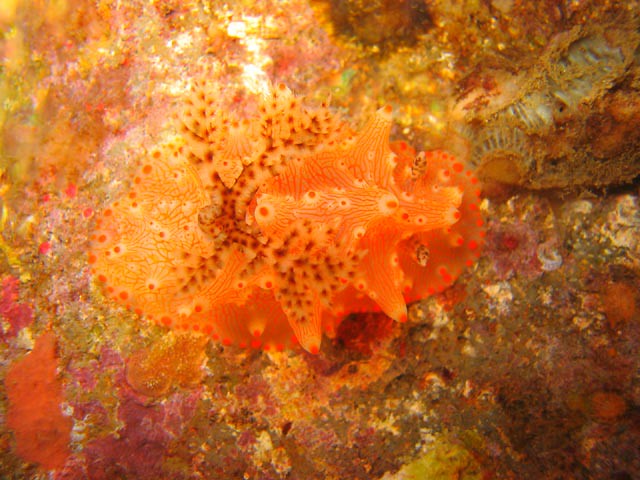The image is an abstract, mystical scene reminiscent of an underwater environment, though it lacks the typical blues and greens associated with the sea. The composition features a mixture of earthy colors, with browns and purples dominating the right side, complemented by a dark cream background and dark tones at the bottom right. In contrast, the left side displays brighter, more vibrant colors with hints of orange, green, pink, and magenta, particularly near the upper left-hand corner. Dots of red are scattered throughout.

In the center of the image, an enigmatic, oval orange form, resembling a sea creature or coral, commands attention. This central figure is adorned with various colored speckles—brown, white, orange—and has protruding sections with leopard-like spots. Some branches extend from this central shape, hinting at a starfish-like form with five appendages. The bottom left edge is rich with reds and oranges, while greens and browns intermingle with purples, contributing to the overall dreamlike quality of the artwork.